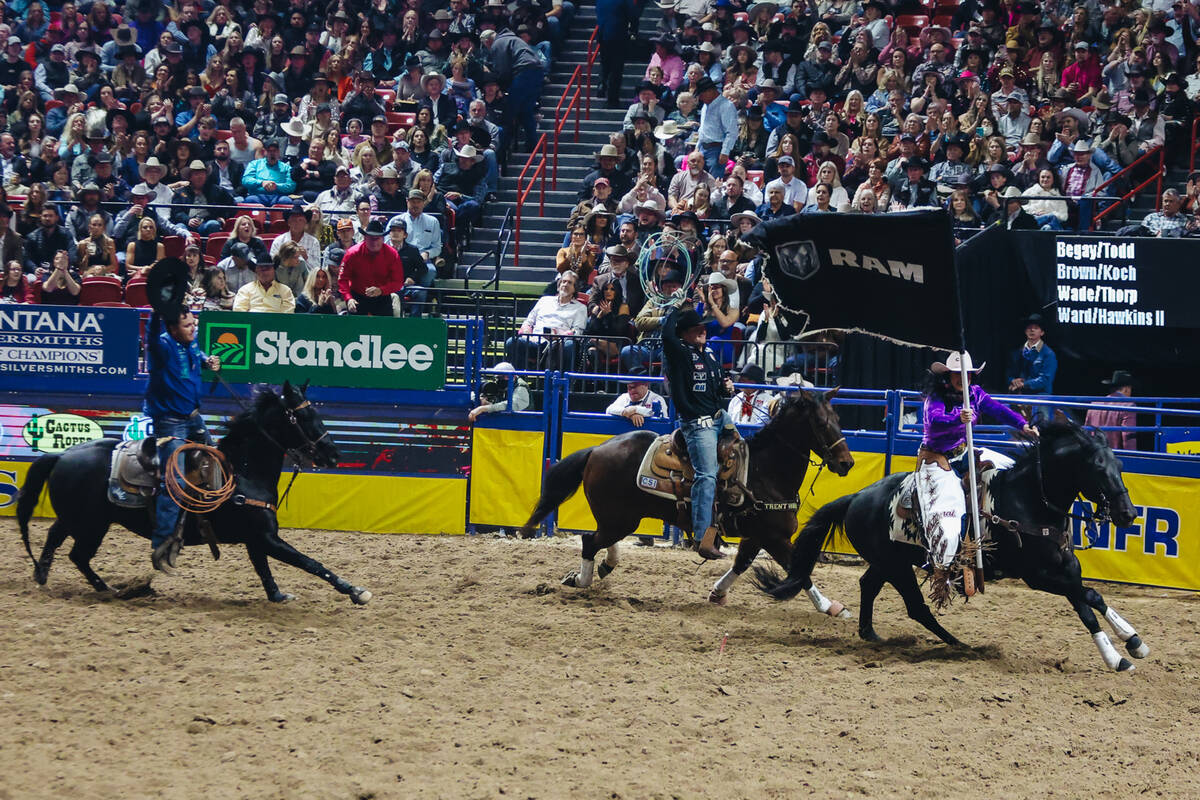In this vibrant rodeo scene, three riders command the dirt arena, each on a majestic horse. The first rider, dressed in a purple shirt and white pants, leads the procession atop a black horse, brandishing a flag proudly displaying the Ram logo. Following closely is a rider on a brown horse, attired in a black shirt with patches and blue Levi jeans, skillfully twirling a lasso in the air. Bringing up the rear is a cowboy on a black horse, lifting his black hat high, clad similarly in a blue shirt and blue jeans. The background is alive with energy, as a packed audience fills the bleachers, their excitement nearly palpable. The scene is framed by a fence adorned with various advertisements, including a prominent one for Stan Lee. To the right of the image, four names—Be Gay Todd, Brown Cock, Wade Thorpe, and Ward Hickens II—are listed, further anchoring this lively moment in rodeo tradition.